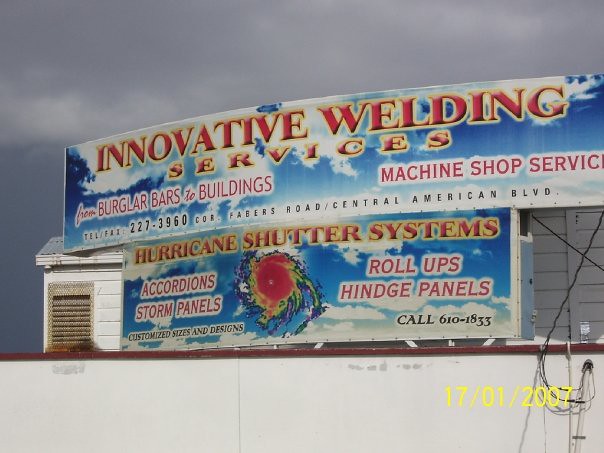The photograph, taken on 17 January 2007 as indicated by the yellow date stamp at the bottom right corner, features a pair of vertically stacked rectangular signs against an overcast sky with portions of a white building visible in the background. The upper sign serves as an advertisement for "Innovative Welding Services," displaying its name in bold red text outlined in yellow, set against a vivid blue sky with white clouds motif. Below the main title, red text on the left and right sides respectively states "From Burglar Bars to Buildings" and "Machine Shop Service," with contact details including "TELFAX 227-396" and the address "Cofammers Road Central America Boulevard" below. The lower sign, carrying the same sky-themed background, promotes "Hurricane Shutter Systems." It features bright red text bordered by yellow, and highlights various products such as "Accordion Storm Panels" and "Roll-Ups Hinge Panels," accompanied by a radar image of a hurricane in the center. Additional service offerings like "Customized Sizes and Designs" are mentioned nearby. The sign concludes with another contact number, "Call 610-1833," in black text.